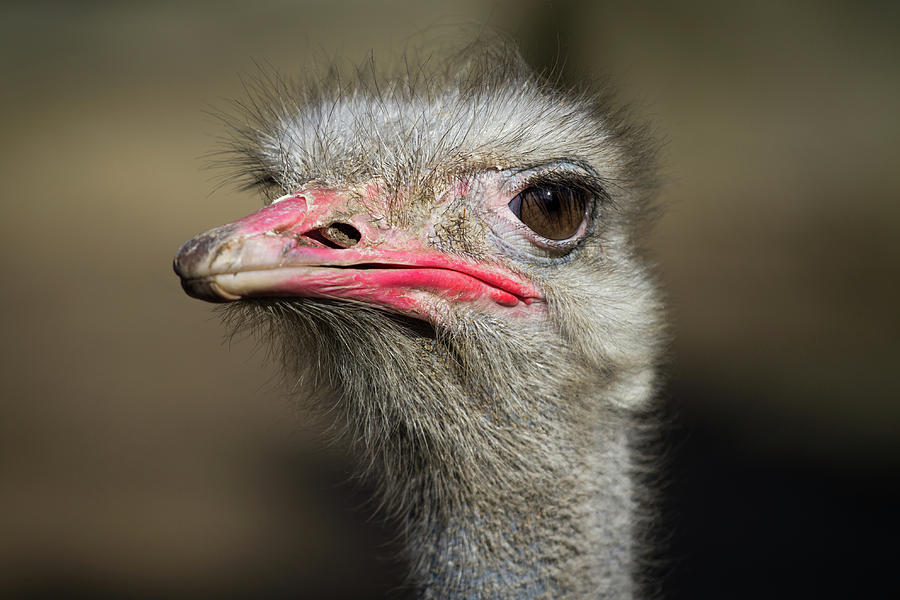The image features a high-definition close-up of what appears to be an ostrich, displaying only the upper neck and head. The background is a blurry mixture of gray and brown, concealing any specific setting. The ostrich is captured with its head turned slightly to the left, presenting one large, dark brown eye with a prominent black pupil and black eyelashes. Its head and neck are covered in medium gray down interspersed with black hairs. The beak, an intriguing mix of colors, is primarily pink with some areas of bright lipstick red and shades of gray at the tip and along parts of the edges. Its beak also features nostril holes. The high-definition quality of the photo highlights every detail, including the texture of its feathers and the subtle nuances of its beak coloring, making it a striking and detailed portrait of the bird.